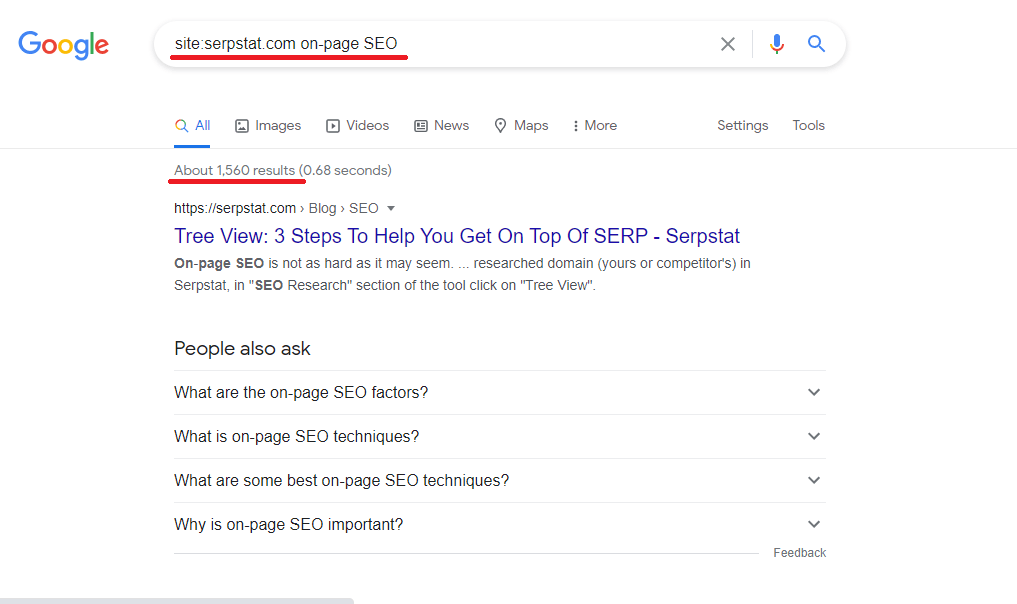A screenshot with a white background displays the Google search results page for "scrpstat.com on-page SEO." The interface highlights include options for images, videos, news, maps, settings (indicated by three vertical dots), and tools. The search yielded approximately 1,560 results, highlighted in red, with the search duration noted as 0.68 seconds.

Prominently featured is a section titled "Three Steps to Help You Get on Top of Scrpstat On-Page SEO." This section reassures users that mastering on-page SEO is not overly complex and emphasizes the importance of researching both your own and competitors' domains. The term "Research" appears in bold, underlining its significance.

A section labeled "SEO Research" is highlighted, with "Tree View" in quotation marks indicating an actionable item within the tool. Additionally, the screenshot includes a "People Also Ask" section with common queries such as "What are the on-page SEO factors?" and "What are on-page SEO techniques?"

Overall, the image captures a detailed and informative snapshot of Google search results focused on optimizing SEO strategies using scrpstat.com.